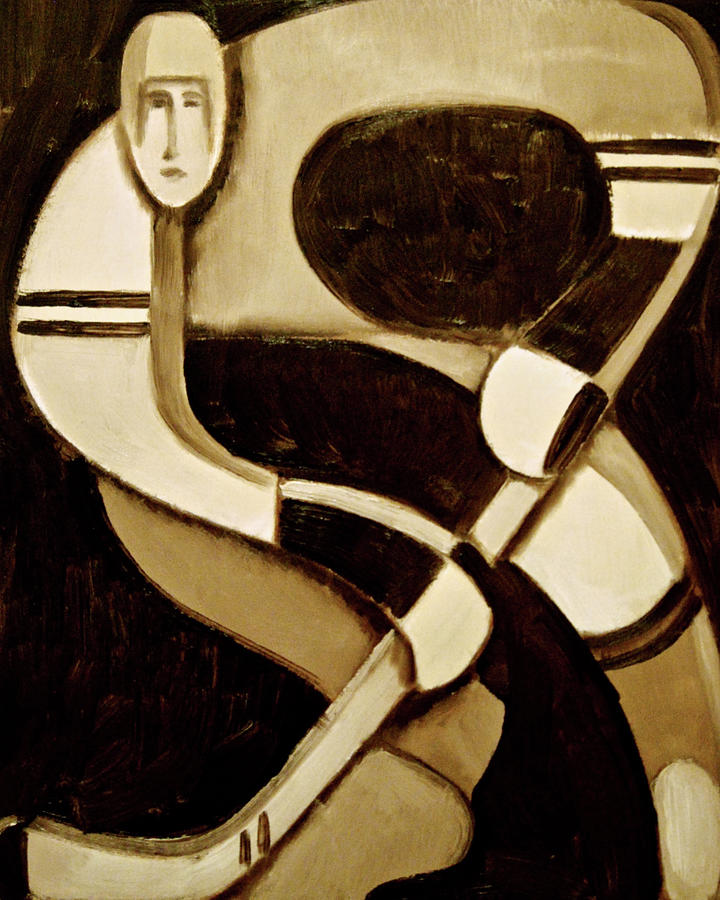The image portrays an abstract artwork of a hockey player in a monochromatic palette, predominantly featuring shades of black, white, and sepia tones. The hockey player is positioned front-facing, with a hockey stick extended towards a puck. Emphasizing fluid motion, the player is rendered with flowing curves that create an almost S-shaped posture. The player's face, with distinctive facial features resembling a carved wooden mask, forms a vertically tall oval situated in the upper left corner of the composition. The background is a solid black, offsetting the hockey player's figure, which is detailed with a jersey bearing two black stripes on each arm and matching socks adorned with a stripe. The brushstrokes are visible, adding texture and depth to the image, giving it a dynamic and somewhat rustic feel.